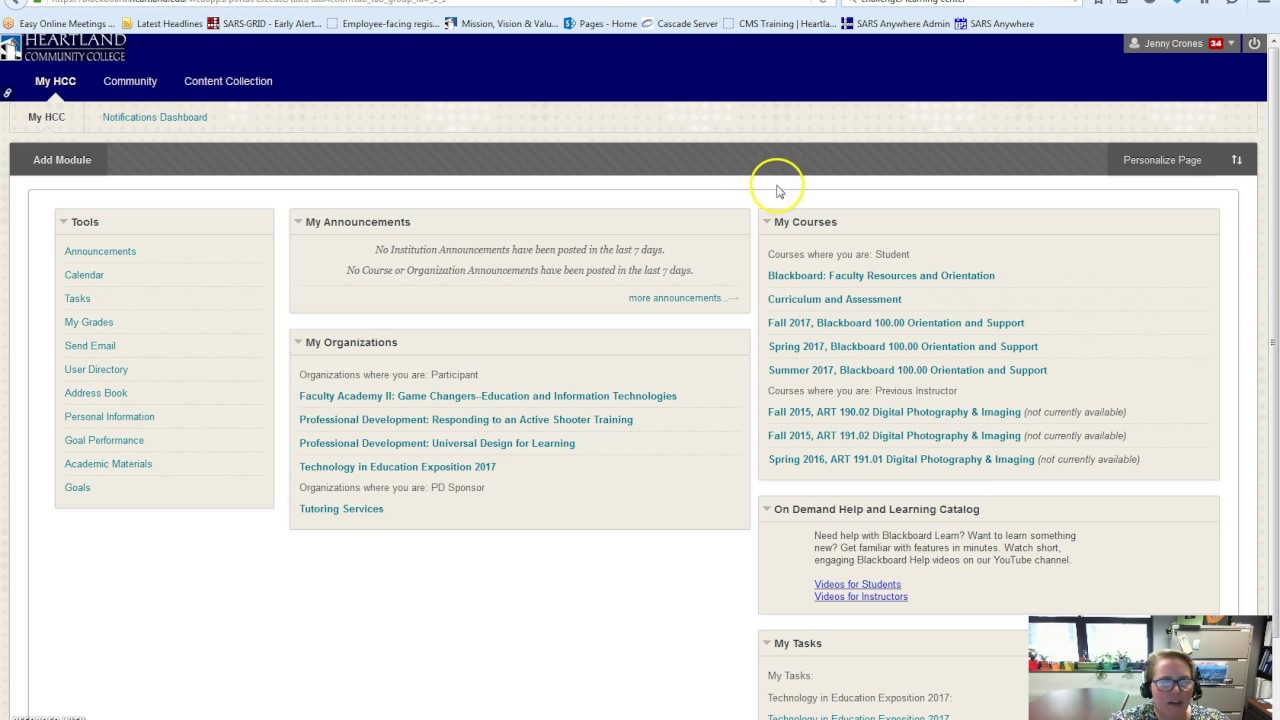This is a low-resolution, blurry screenshot of an Internet Explorer window, which suggests it is an older image. At the top of the window, there is a blue bar with several unreadable bookmarks. Below this bar, a darker blue rectangle on the left corner displays "Heartland Community College" with "MyHCC" highlighted in white font beneath it. To the right, it reads "Community" and "Content Collection."

The area below this contains a beige rectangle labeled "MyHCC Notifications Dashboard." Following this, a gray rectangle features the text "Add Module" alongside some other unreadable text. Beneath this section, a white rectangle is present with a yellow circle in the middle, where the computer cursor is located. 

Further down, there are several beige squares with various menus in black font. The leftmost menu, labeled "Tools," includes options such as Announcements, Calendar, Tasks, My Grades, Send Email, User Directory, Address Book, Personal Information, Goal Performances, Academic Materials, and Goals. To the right of this, additional categories listed in black font include "My Announcements," "My Organizations," "My Courses," and "On Demand Help and Learning Catalog."